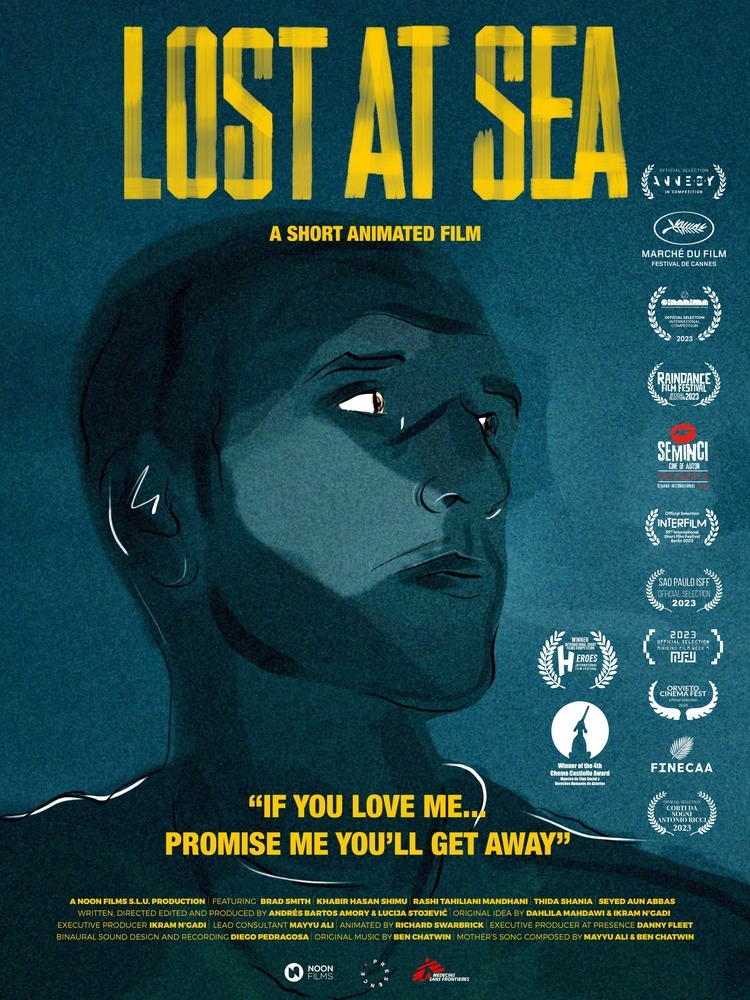This movie poster for "Lost at Sea," a short animated film, features striking use of color and design elements. Dominated by a dark bluish background with shades of light blue, the top of the poster boldly displays the film's title "Lost at Sea" in large yellow text. Below the title, it reads "a short animated film" in smaller text. 

The central focus of the poster is an animated headshot of a man, who is silhouetted in dark bluish-gray with subtle lighter shades adding contrast. His eyes are white with small brown pupils, and white lines delicately outline his ear, collar, and neck area. The man's face, depicting him looking slightly to the right, adds a mysterious and reflective tone to the poster.

At the bottom of the poster, in yellow text, a poignant quote reads, "If you love me, promise you'll get away." Below this, the credits, listing the directors, producers, and other key contributors, are displayed in yellow text as well. The bottom section also features the production company's name, Noon Films, in white text. A circle symbol and a red icon are present, although the text near these symbols is indistinct.

To the right of the poster, a collection of logos represents various film festivals and organizations such as the Sundance Festival, Interfilm, Raindance Film Festival, and others. These logos, which include Sao Paulo, ISFF, and Marche du Film Freecans, are arranged in white, emphasizing the film's recognition in the independent movie circuit.